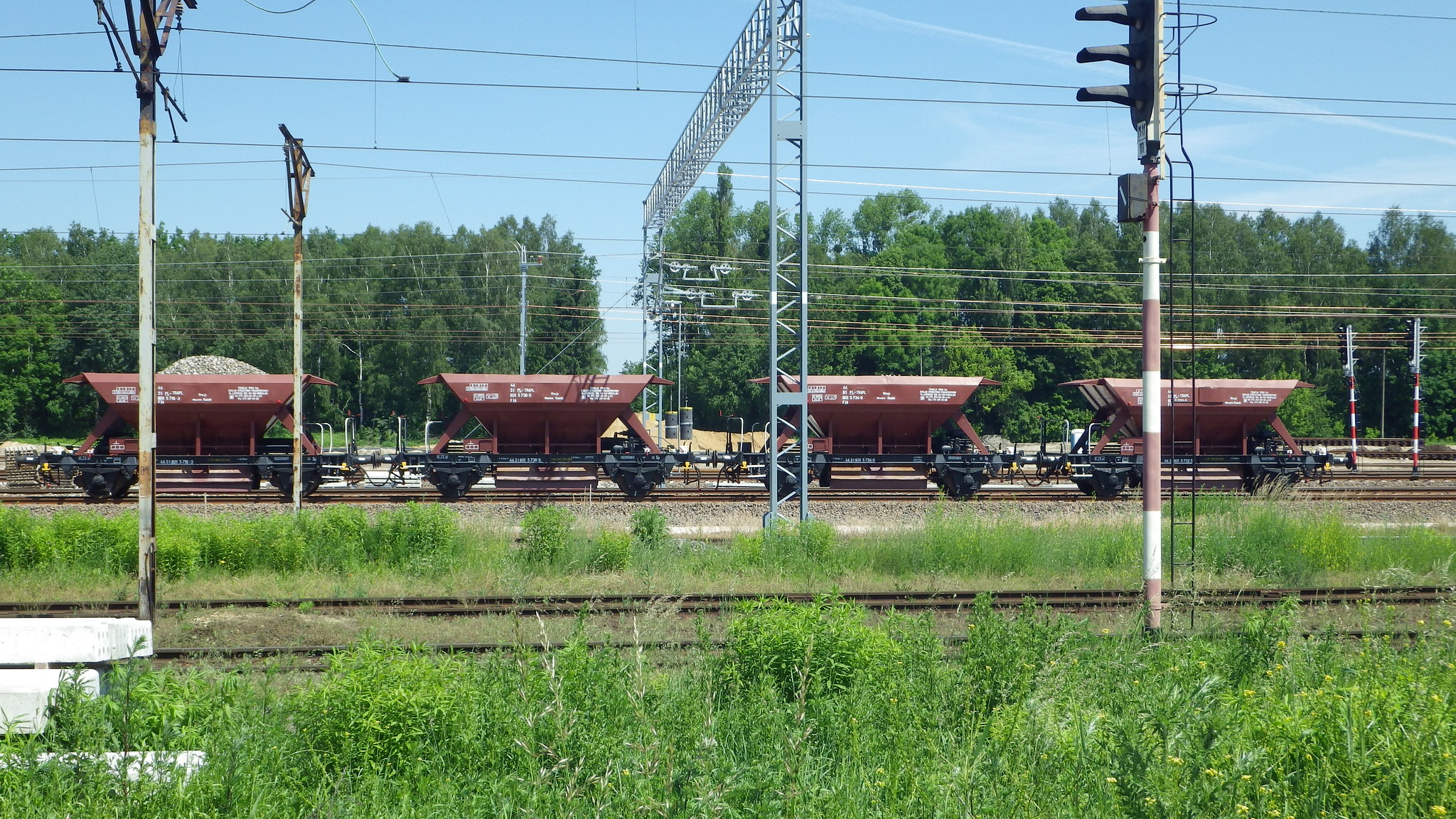The image depicts a clear, sunny day with a striking blue sky dotted with faint white clouds. The background is dominated by a lush line of green leafy trees, with a small break in the center revealing more sky, while the foreground is filled with tall green grass. A railway track cuts through the scene, flanked by more grass and a slight hill of gravel. There are four connected carriages or loaders, resembling clay-colored buckets on wheels, positioned on the track. The front loader, on the far left, contains a mound of gravel, with small rocks plainly visible, while the other three appear empty. Interspersed throughout the image are grey power poles, some showing signs of rust, and the bottom right corner features a distinctive white and red pole with a black-topped robot-like device affixed to it and a staircase behind it. Additionally, there are white concrete slabs at the bottom left of the image, and the scene is lined with various plants, echoing the verdant surroundings.